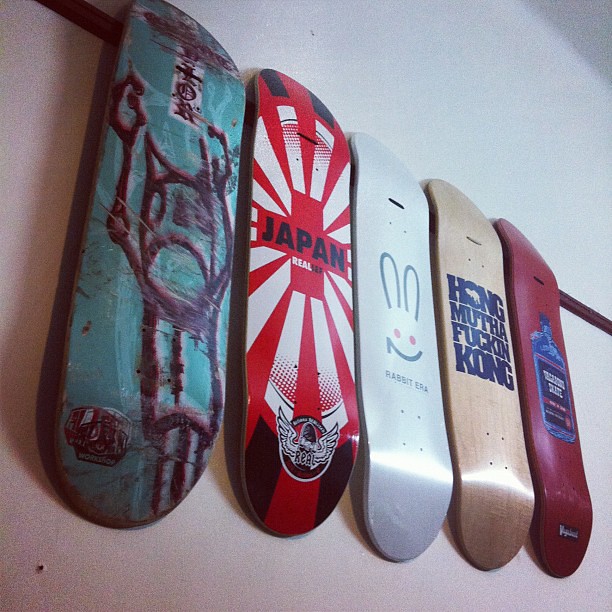The photograph showcases five skateboards hanging vertically on a wall, each with distinctive graphical designs. From left to right: The first skateboard is light teal with a black silhouette character that has raised hands, horns, and appears to be screaming. The second skateboard is predominantly red with white sun rays and the text "Japan" at its center. The third skateboard is white, featuring a cartoon bunny with pink eyes and black outlines for the ears and mouth, alongside the caption "Rabbit ESA." The fourth skateboard displays a natural wood color and bears the text "Hong motherfucking Kong" in bold black letters. The fifth skateboard is solid red with an indiscernible design. These skateboards are attached to a wooden strip mounted on the wall, possibly within a house or similar indoor setting.